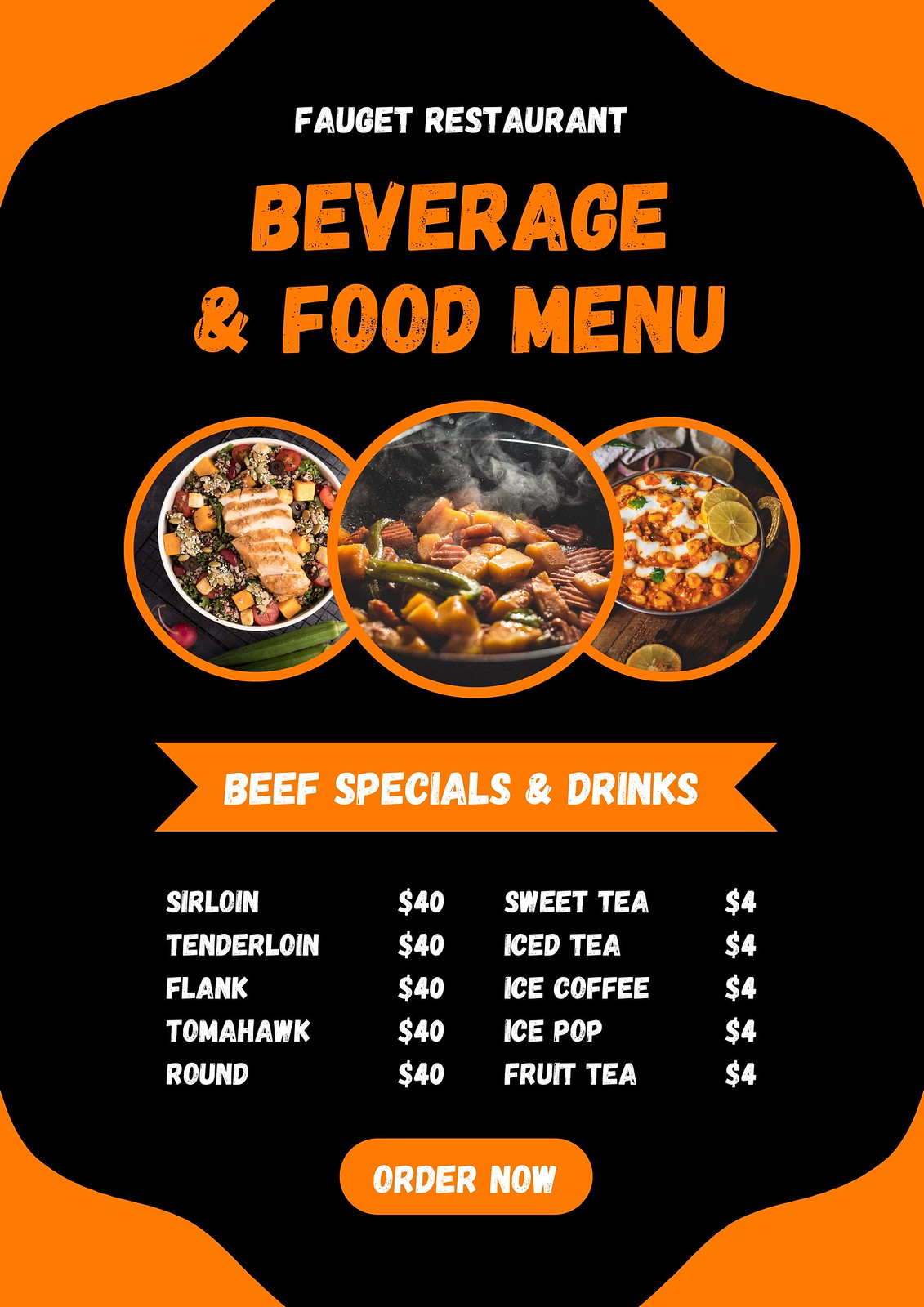The graphic advertisement prominently features a black background with a vivid orange base, designed to showcase a restaurant menu. At the top, the title reads "Forget Restaurant" in white lettering and "Beverage & Food Menu" in orange lettering, both with subtle black artifacts giving them a textured look.

Beneath the title, three orange circles capture attention with photographs of appetizing dishes. The left circle displays a bowl of sliced chicken and an assortment of vegetables. The middle circle shows a steaming black bowl filled with green and orange vegetables. The right circle provides an overhead view of a black bowl containing food smothered in a reddish-orange sauce, garnished with lemon slices.

An orange banner below these images announces "Beef Specials & Drinks" in white lettering. Listed underneath are beef dishes each priced at $40: Sirloin, Tenderloin, Flank, Tomahawk, and Round. The menu also highlights a variety of beverages, each marked at $4: Sweet Tea, Iced Tea, Iced Coffee, Iced Pop, and Fruit Tea.

At the bottom of the advertisement, an orange horizontal oval presents a call-to-action with "Order Now" boldly written in white letters.